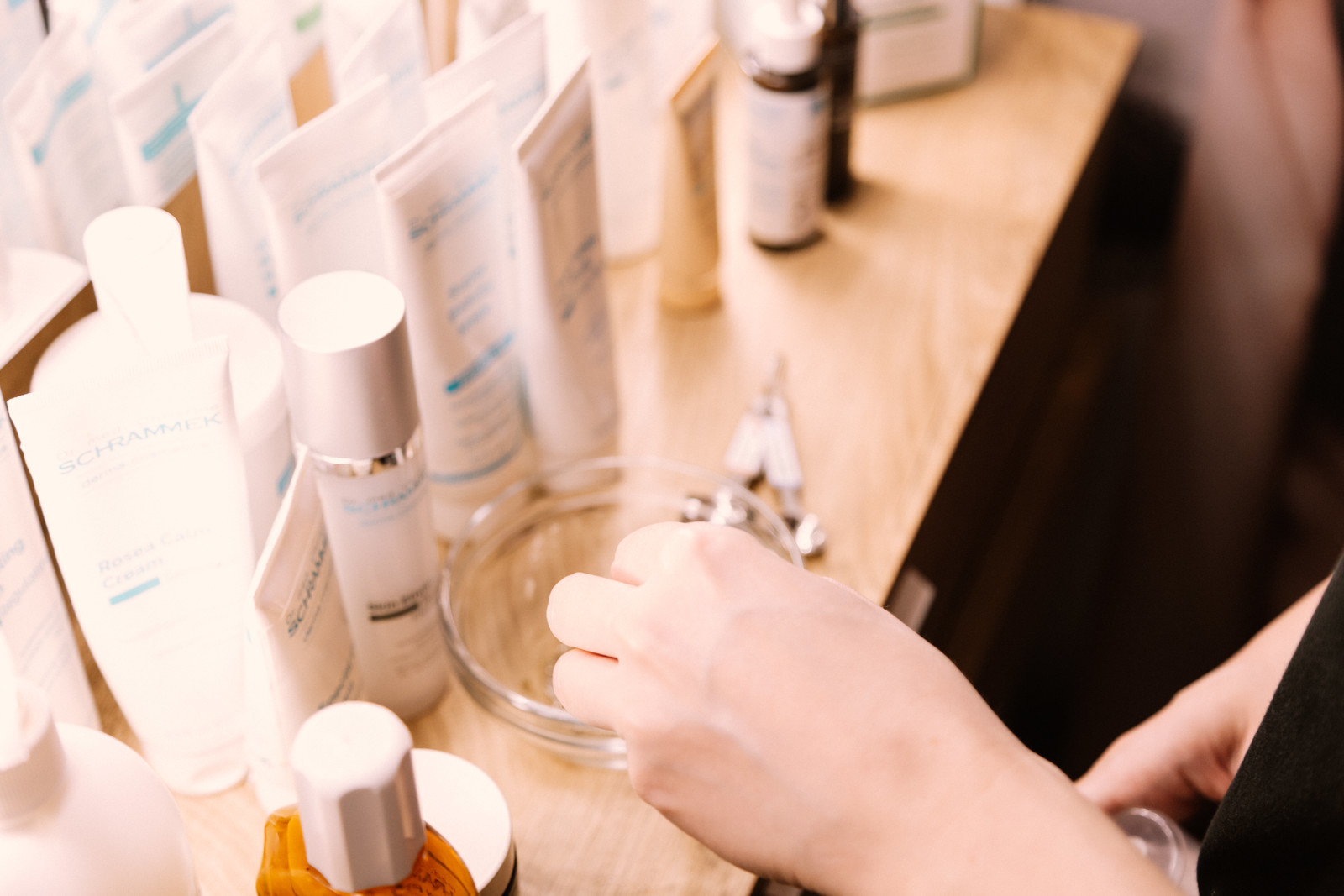This image depicts a serene setting likely intended for a facial treatment, focusing on a light wooden countertop adorned with various skincare products. A woman's left hand is seen reaching into a clear glass bowl, while her right hand is held closer to her body, just partially visible. The countertop is organized with an assortment of skincare products, predominantly from the Dr. Schrammich brand. 

To the left side of the image, there are multiple product containers. The lineup begins with two tubes of different sizes, followed by two bottles. To their right, four more upright tubes are displayed, with three additional tubes further along. All these containers are white with blue lettering, contributing to a clean and professional aesthetic. Toward the back of the countertop, details become blurred, but you can discern another small yellow tube and a small bottle featuring white labels with blue text. Adjacent to the glass bowl is a tiny metal instrument, presumably a tool used in the facial treatment process.